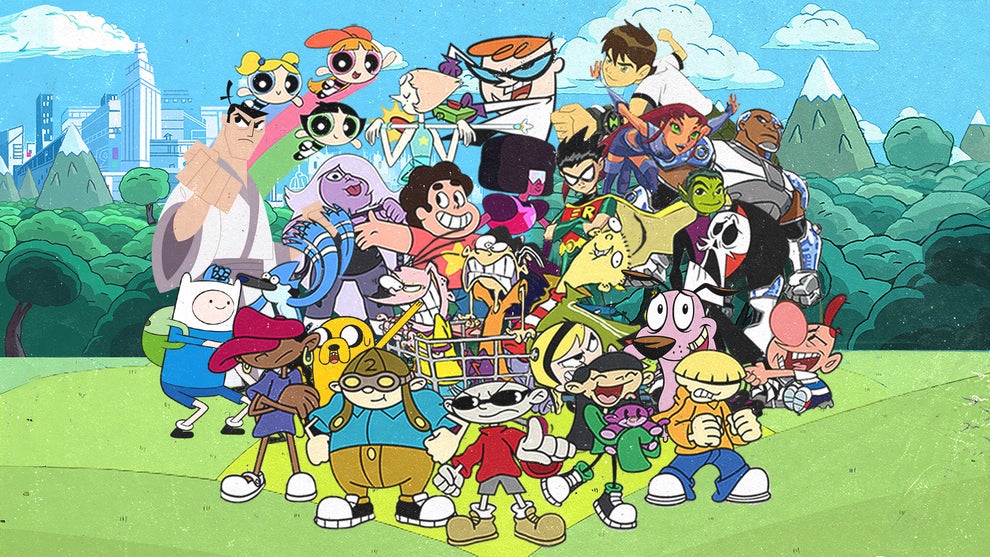This image is a vibrant, detailed cartoon drawing featuring a diverse ensemble of about 40 different cartoon characters, many of which are recognizable from popular children's shows on Cartoon Network. The scene is set outdoors with a lush lime-green grass field in the foreground, backed by a skyline that includes a cityscape to the left, a range of mountains in the middle, and trees with rounded leaves. Overhead, the sky is dotted with clouds.

Prominently featured are iconic characters such as the Powerpuff Girls, who appear to be flying in the sky. Also noticeable are Courage the Cowardly Dog, characters from Billy and Mandy, Ed, Edd n Eddy, Codename: Kids Next Door, Adventure Time, Dexter's Laboratory, Ben 10, Teen Titans (with a clear nod to Robin from Batman and Robin), Samurai Jack, Steven Universe, and Regular Show. Among these characters is also a green-faced alien and a girl with a purple face and light purple hair. Additionally, there's a guy with an oval-shaped head, wearing oval sunglasses, a red turtleneck, and gray shorts, reminiscent of Stewie from Family Guy.

All these characters are grouped together in a lively collage-like arrangement in the middle of the scene, creating a bustling, celebratory atmosphere against the rich, diverse backdrop of natural and urban elements.